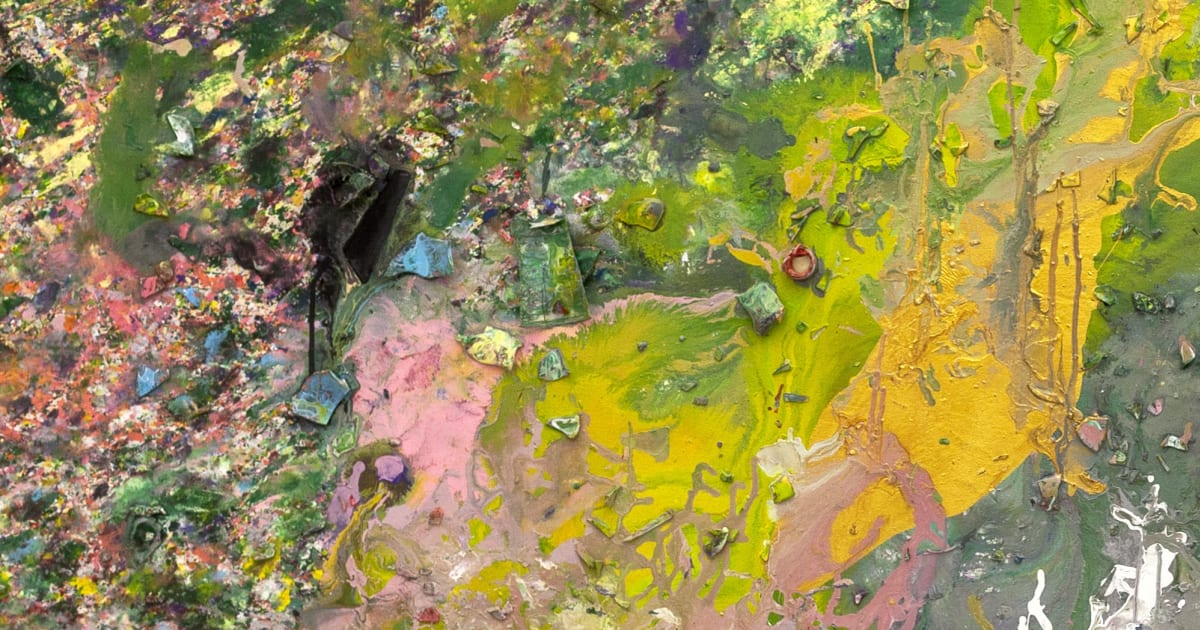This oil painting presents an abstract and richly textured scene that evokes a sense of wild, untamed nature. At first glance, the image remains elusive, but upon closer inspection, it reveals a dynamic interplay of colors and textures. The bottom right corner features a patch of white, transitioning into an area of muddied olive green, which occupies about a tenth of the painting. Above this, vibrant strokes of bright yellow and yellow-green are thickly applied, creating areas of impasto that give the painting a tactile, almost three-dimensional quality.

Scattered throughout the composition are fragments of blue-colored debris, possibly broken pottery, adding an unexpected material element to the painting. On the left third of the canvas, the brushstrokes come together to suggest a flower scape, a burst of splotchy yet harmonious colors. This section is alive with shades of pink, green, blue, yellow, and purple, depicting an abstract representation of wildflowers in a natural setting. The overall effect is a vivid, chaotic, yet beautiful portrayal of a flower-laden meadow, rendered in a splashy, expressive manner.